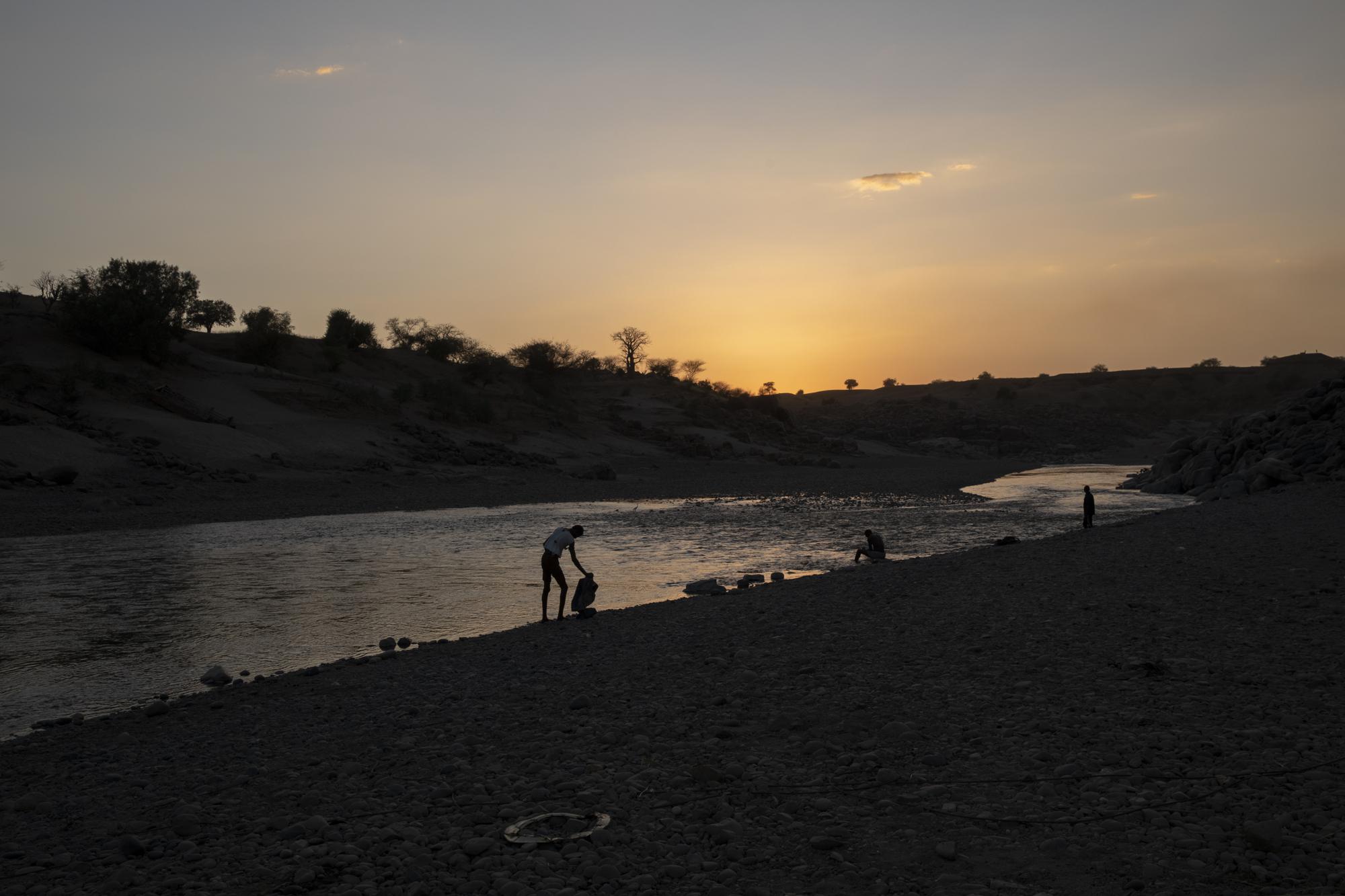The image captures an outdoor scene at dusk or dawn, with the sun positioned just below the horizon. The sky is illuminated in a gradient of gold, orange, and pink hues, with a few sparse clouds—a small one near the center and another in the top left corner. Just beyond the horizon, a line of hills, some with small trees, gently descend towards the river. In the foreground, a river courses from the left side diagonally upwards toward the right, making a turn before it reaches the edge of the picture. On its banks, a mixture of gravel and rocks is visible. Three individuals are seen near the river: one person on the left stands with their feet in the water, holding a backpack; the second individual, closer to the right, sits in the water; while the third person stands on the far right bank, possibly engaging with the river scene. A bridge is visible in the distant background, over which the dusky sky casts an array of vibrant colors. The overall aesthetic is primarily in shadow, creating a striking contrast with the golden horizon.